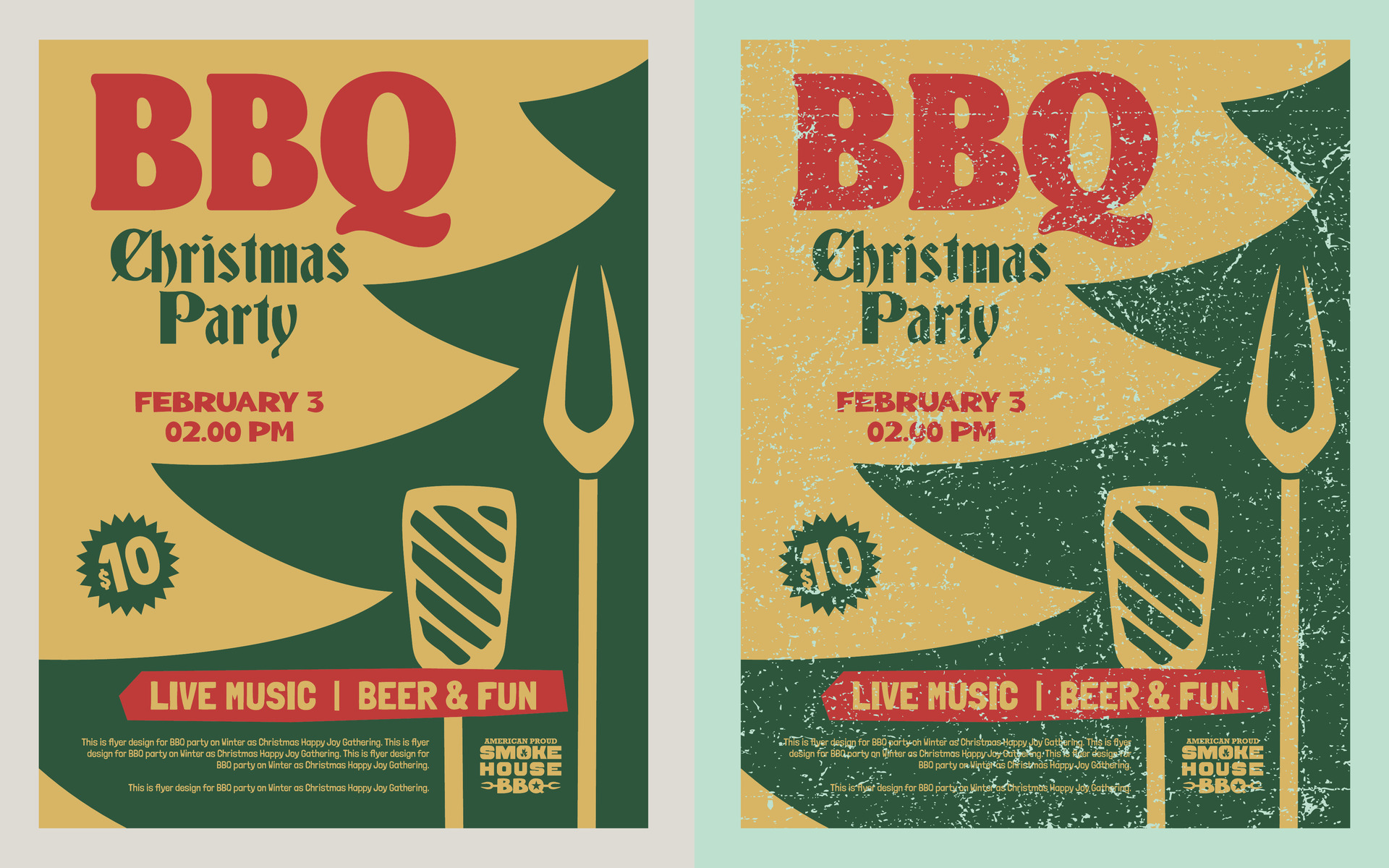This image displays two advertisements for a "Barbecue Christmas Party" scheduled for February 3rd at 2 p.m. with an entry fee of $10. Both posters, set against a mustard yellow background, prominently feature the event details in red and green, evoking Christmas colors. The posters highlight "Live Music, Beer, and Fun" at the "American Proud Smokehouse BBQ" venue. The central graphic prominently consists of the silhouette of a pine tree adorned with BBQ utensils, including a fork and a turner, emphasizing the festive and culinary theme. Notably, one poster appears brand new with a light green outline, while the other, outlined in gray, looks worn and weathered, possibly due to being exposed to elements. The advertisements have small, indistinct print, likely placeholder text describing the event as a winter holiday gathering. The left poster retains a pristine look, whereas the right one has a grungy, distressed texture, indicative of wear and tear.